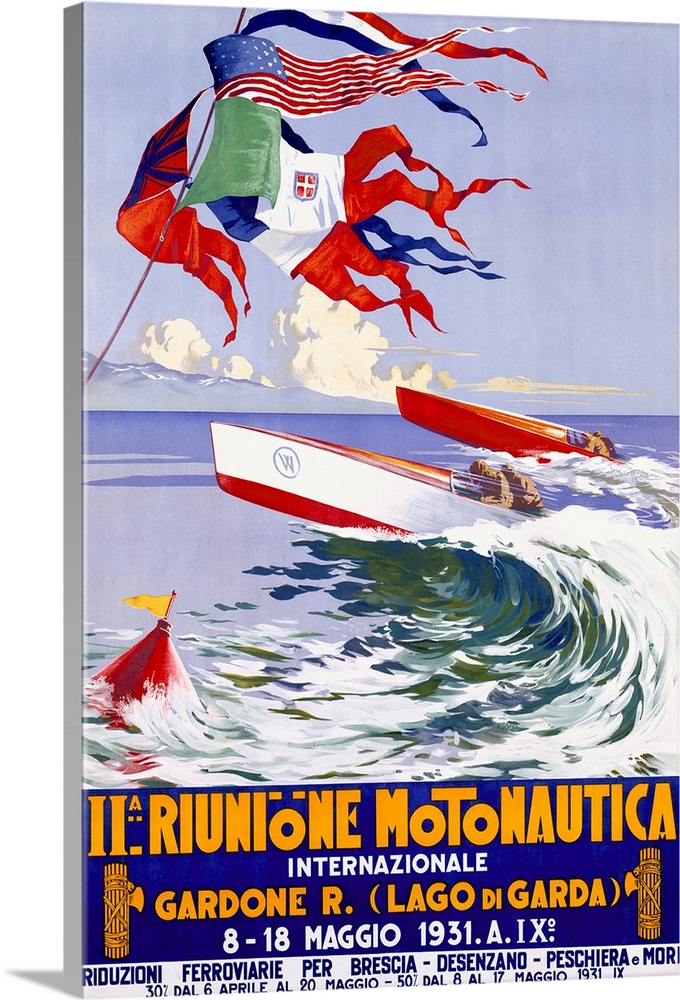This is a vibrant, upright rectangular poster, primarily written in Italian, promoting the "Riunione Motonautica Internazionale Gardone Lago di Garda 8-18 March 1931," listing several cities below the event details. The painting depicts a dynamic boat race on Lake Garda, featuring two speeding raceboats—one white with red trim and the other predominantly red—racing from right to left, creating intense, cresting waves in dark blue and green hues. A notable buoy with a yellow flag is also visible in the water. In the background, a clear sky is punctuated by several national flags, prominently the American flag, the Italian flag with its red, white, and green colors, the French flag, likely the British flag, and potentially the Czech flag. The overall imagery and bright colors convey the excitement of an international boat racing event.